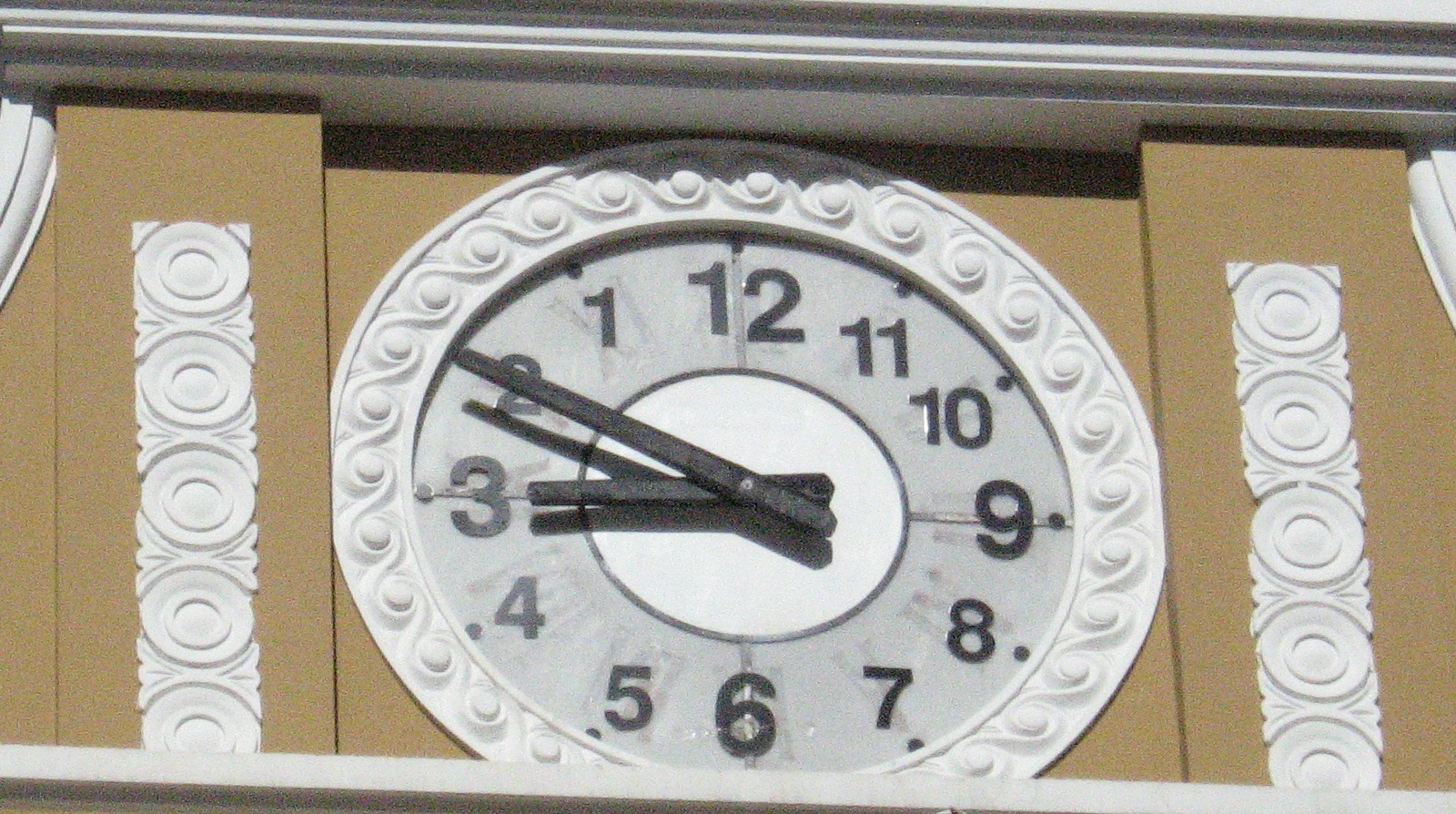A striking clock is prominently displayed in a large public space. The clock features an inlaid white marble face surrounded by ornate Roman-style decoration on a circular frame. The numbers on the clock face are of particular interest: the 12, 3, 6, and 9 are larger than the other numerals, but they are arranged in a counterclockwise manner, giving the appearance that the image is reversed. The smaller ancillary numbers—1, 2, 4, 5, 7, 8, 10, and 11—are meticulously placed in between. Bold black minute and hour hands point to 3:10 in this unusual, yet captivating timepiece. The grandeur and design suggest it could be a centerpiece in a town square or a similar public venue.